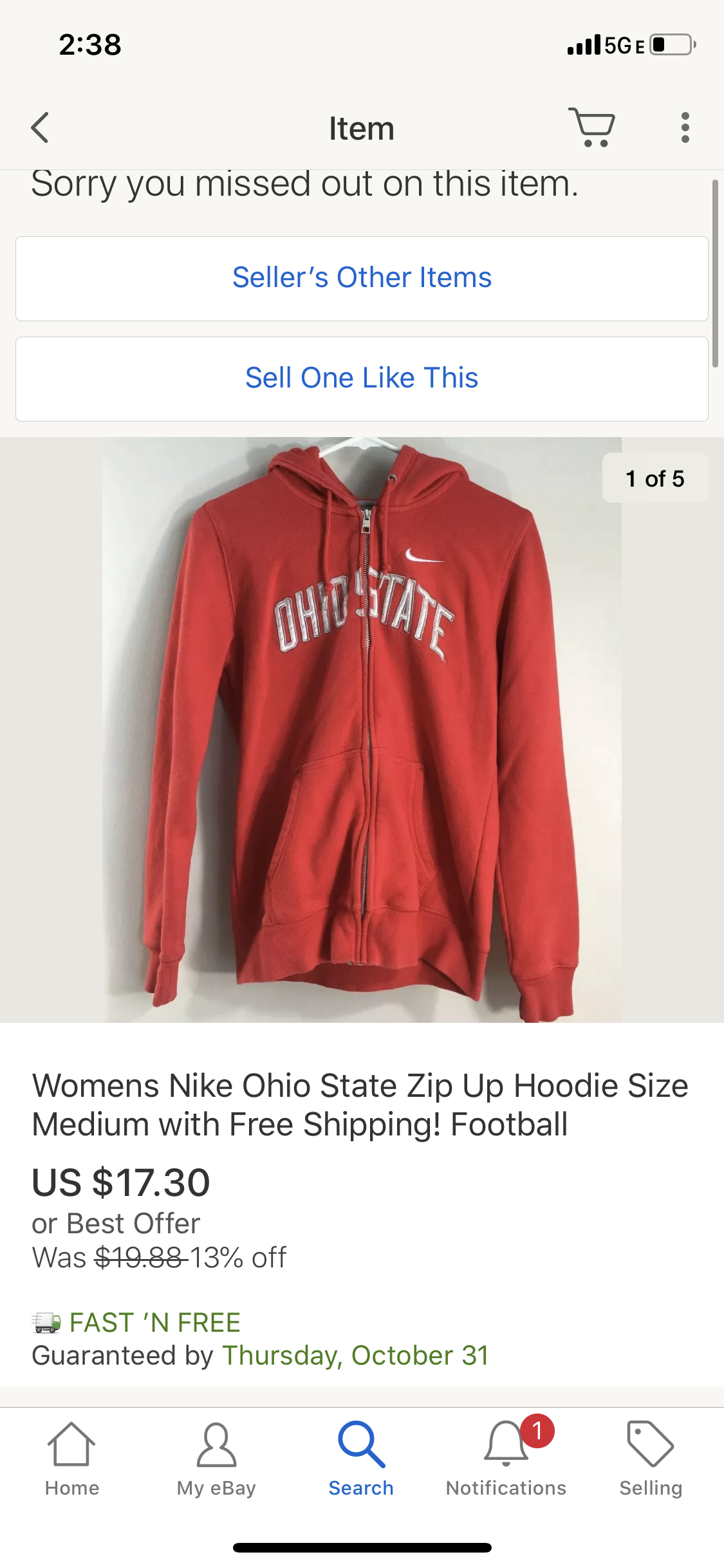The image is a color screenshot taken on a mobile device, likely an iPhone, showcasing an eBay listing for a women's Nike Ohio State zip-up hoodie, size medium, available for $17.30 or best offer. The screenshot displays a message at the top saying, "Sorry, you missed out on this item," with links below it to view the seller's other items or to sell a similar item. The hoodie, prominently shown in the center, features the words "Ohio State" in white, accompanied by a description indicating free shipping and a 13% discount off the original price of $19.88. Additional details include the promise of a fast and free delivery by Thursday, October 31st. Navigation buttons for home, my eBay, search, notifications, and settings are visible at the bottom of the screen, confirming the listing is from the eBay app. The colors in the screenshot include tan, black, white, blue, red, and green.